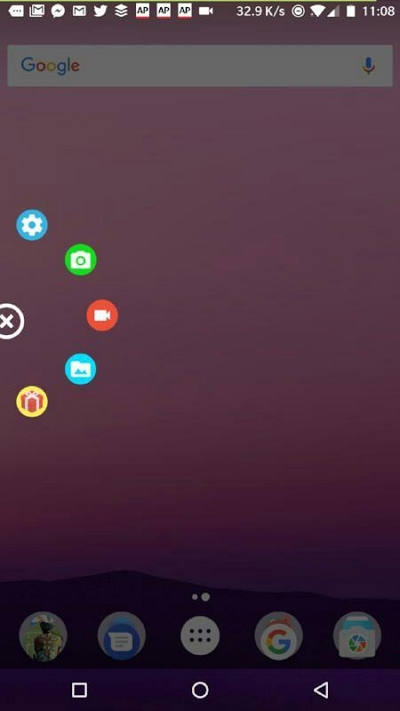The image appears to be a screenshot of a smartphone home screen with a purple background. At the top of the screen, there are various notification icons, including Gmail, Facebook Messenger, and Twitter. Additionally, it shows a cell signal indicator with moderate strength, full Wi-Fi signal, full battery level, and the time displayed as 11:08 AM. Below these notifications is a search bar with the Google logo and a microphone icon beside it.

In the bottom left corner, there's an icon of a person, likely representing a user profile or contacts. Next to it is a folder containing several applications. This is followed by a square icon, a circle icon, and a sideways triangle icon pointing left, which could represent navigation buttons.

In the center of the screen, towards the left side, there are several application icons arranged in an arc. These include a blue circle with a gear (likely settings), a green camera icon, a video icon, a folder with a photo, and a yellow circle with a present box. There is also an icon labeled "32.9 KSSI."

The bottom section of the screen is black, possibly indicating the absence of a navigation bar or a section reserved for additional controls.